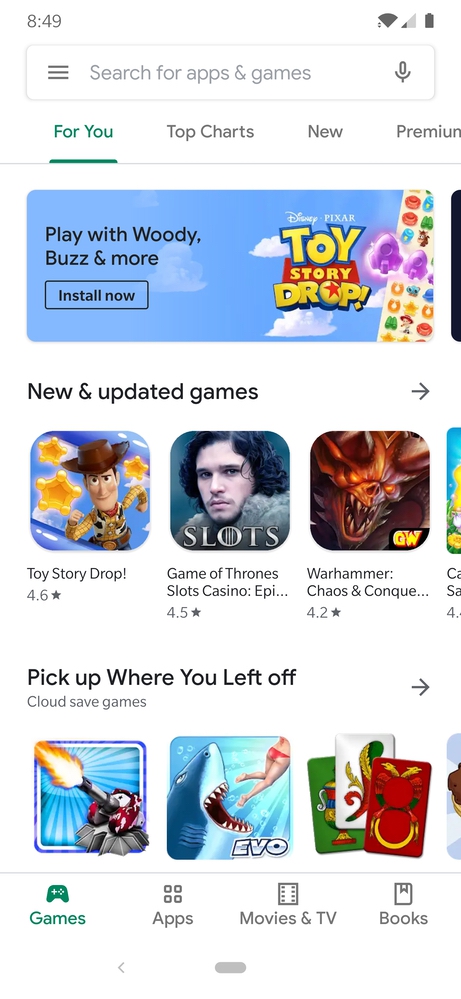This screenshot from an Android device showcases the Google Play Store interface. The background of the Play Store, as well as the notification bar, is predominantly white. At the very top, the notification bar displays the time, which is 8:49 AM, on the left-hand side. To the right, it shows the Wi-Fi signal, cellular signal, and battery indicators.

Directly below the notification bar, a horizontal search bar is prominently positioned, allowing users to search for games and apps. Underneath this, a menu comprising four options—'For You,' 'Top Charts,' 'New,' and 'Premium'—is arranged horizontally. The 'For You' section is currently in view.

Beneath the menu, a rectangular banner features an advertisement for the 'Toy Story Drop' app with the tagline "Play with Woody, Buzz, and more. Install now." Moving further down, a section titled 'New and Updated Games' presents a list of various games. The first game listed is 'Toy Story Drop,' followed by 'Game of Thrones: Sloth's Casino,' and 'Warhammer: Chaos and Conquest.' Each game entry includes a small icon or logo representing the game.

The next section, titled 'Pick up where you left off,' displays a list of games that the user has previously played or is currently playing. 

At the bottom of the screen, there are navigation options to switch between different categories within the Play Store: 'Games,' 'Apps,' 'Movies & TV,' and 'Books.'